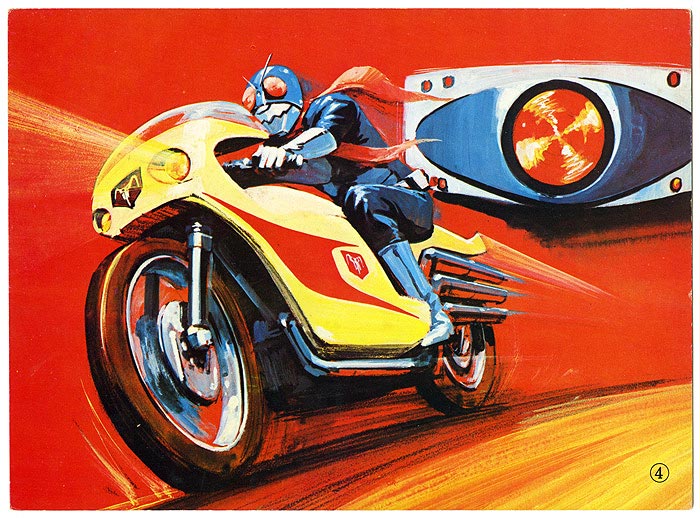The image is a highly detailed comic book-style illustration depicting a bug-themed superhero, possibly female, on a brightly colored yellow motorcycle with red accents. The superhero is dressed in a dark navy blue costume with tall blue boots, a red cape flowing behind, and a blue mask with prominent red circles for eyes, resembling the face of a fly with antennae. The motorcycle, adorned with a red logo and featuring a bug gun on the side, appears to be speeding down a yellow road. The background is entirely red, suggesting urgency or danger, and includes a detailed sensor-like graphic on the right, possibly indicating intelligence or mission data. The composition suggests high-speed motion, accentuated by thin wheels and dynamic lines emitting from the motorcycle's headlight. In the bottom right corner, among this vivid scene, a small black number four enclosed in a circle stands out.